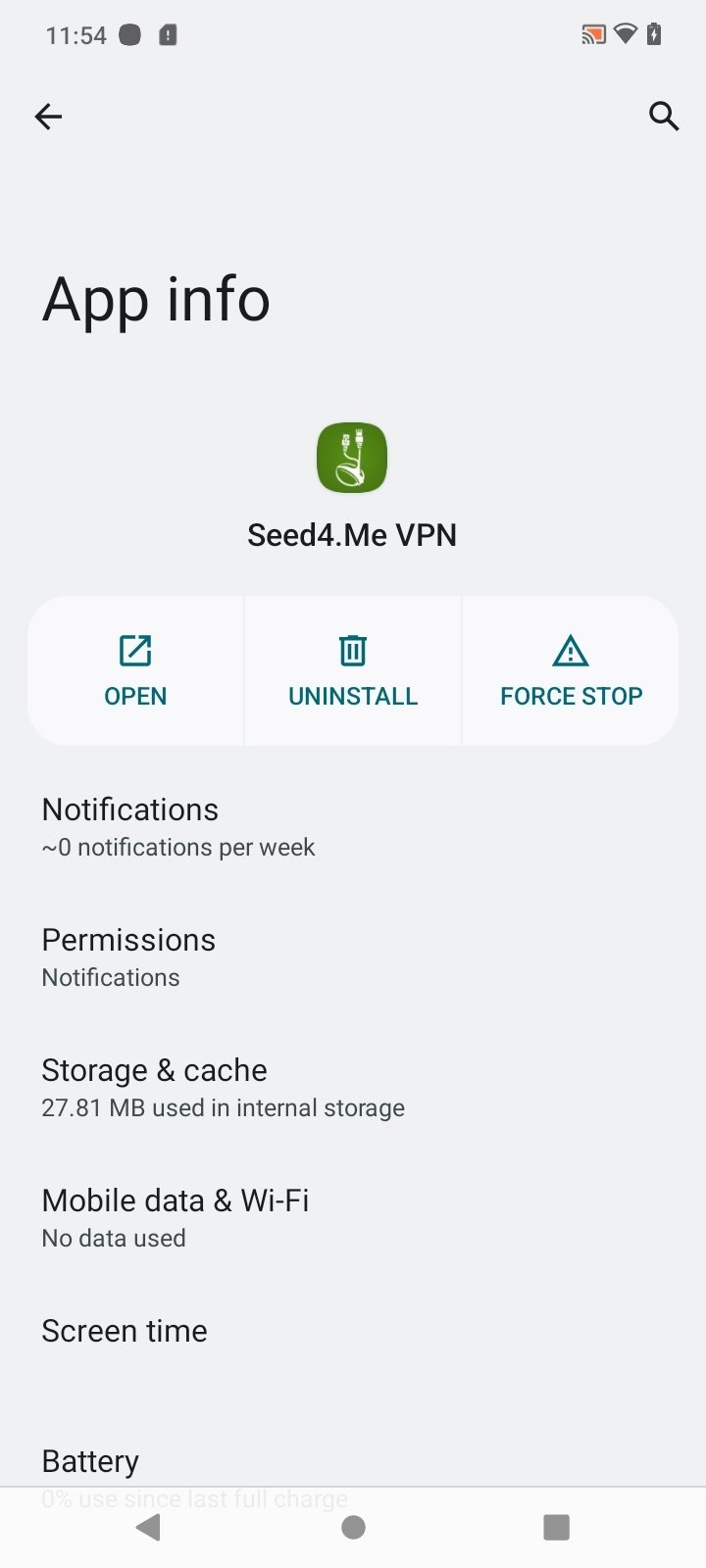This is a detailed description of a smartphone screenshot displaying the information screen of a specific app. At the very top, there is a timestamp showing "11:54" and two icons; one is an indistinguishable black square, and the other is a white exclamation mark inside a tag, likely indicating a warning. To the right of these icons, there is a Wi-Fi symbol, a battery icon, and an RSS feed icon. Below this top bar, on the left-hand side, there is a left-facing arrow, and on the right-hand side is a magnifying glass icon symbolizing search functionality.

The main header of the screen reads "App Info." Directly beneath this title is the app’s logo, which is green and resembles a USB cord. The app name, presented below the logo, is "Seed4.me VPN." Following this are three actionable tabs labeled: "Open," "Uninstall," and "Force Stop."

Detailed information about the app is listed in a vertical order starting with "Notifications," showing "0 notifications per week." The following section is "Permissions" and "Notifications," however, specific details are not provided. Next is "Storage and Cache," with the app using "27.81 MB" of internal storage. The "Mobile Data and Wi-Fi" section states "No data used." "Screen Time" is mentioned next, but specific details are not provided. Lastly, there is a "Battery" section, though no details are given here either.

At the very bottom of the screen, there is a navigation bar containing a left-facing arrow, a home button, and a stop button.